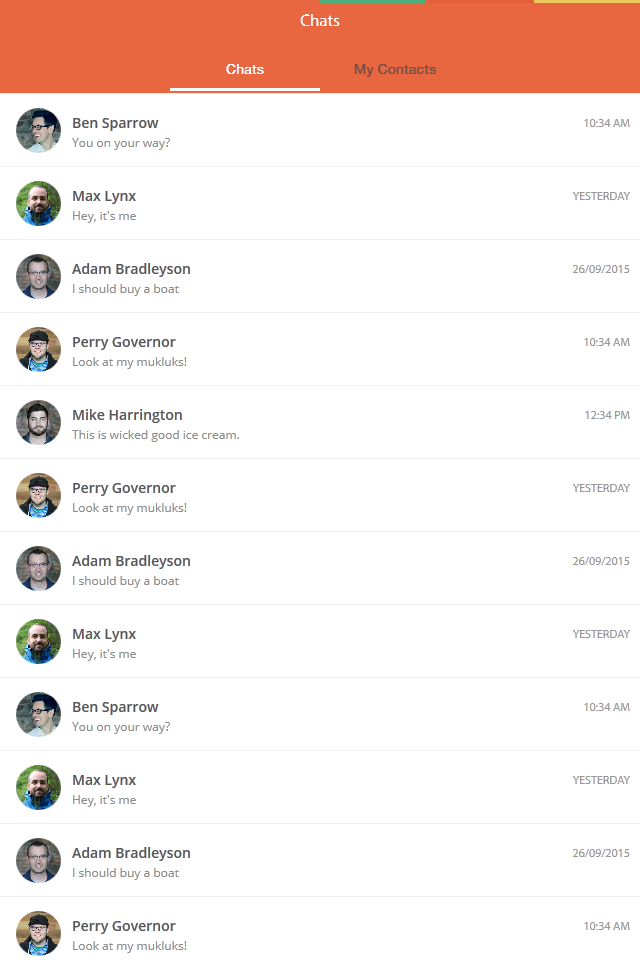The image appears to be a screenshot of a messaging app interface. The top section features an orange header with white text, displaying the current tab "Chats." The inactive tab, also labeled "Chats," is gray, showing a clear visual distinction between the active and inactive sections. At the top right corner, there is a three-color indicator composed of equally-sized green, orange, and yellow lines, each about three pixels thick, matching the orange shade of the header.

Below the header, the interface is divided by thin gray lines into separate sections, each listing individual chats. The background of these sections is white, while the text is gray, maintaining a minimalistic and clean appearance. On the left side of each chat entry, there are avatar images of the chat participants, depicting white men in their 30s or 40s.

To the far right of each chat entry, there are time stamps indicating when the messages were sent. The notable names in the chat list include Ben Sparrow, Max Links, Adam Bradleyson, and Perry Governor, each seemingly repeating the same messages in their respective sections.